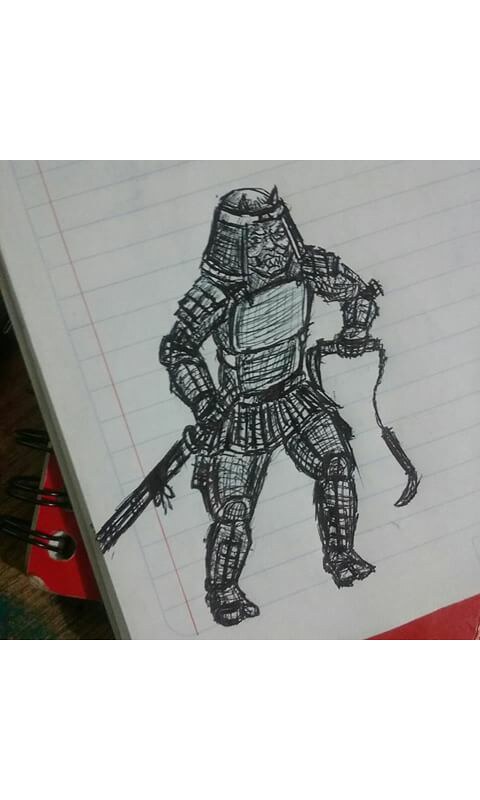In this detailed sketch, a character is illustrated on a white notepad. The bottom left corner reveals a background that resembles light brown flooring, heavily shadowed to appear dark brown. Partial view of the notepad's edge shows three black rings binding it, with a red cover peeking through. The character is fully sketched with both legs visible. The torso is predominantly gray with significant black shading. The character's left hand wields a sword, while the right hand appears to hold either nunchucks or a bow. The face, monstrously illustrated, features two ominous horns protruding from the top of the helmet. The entire sketch employs shades of gray and black, creating a stark, dramatic effect.